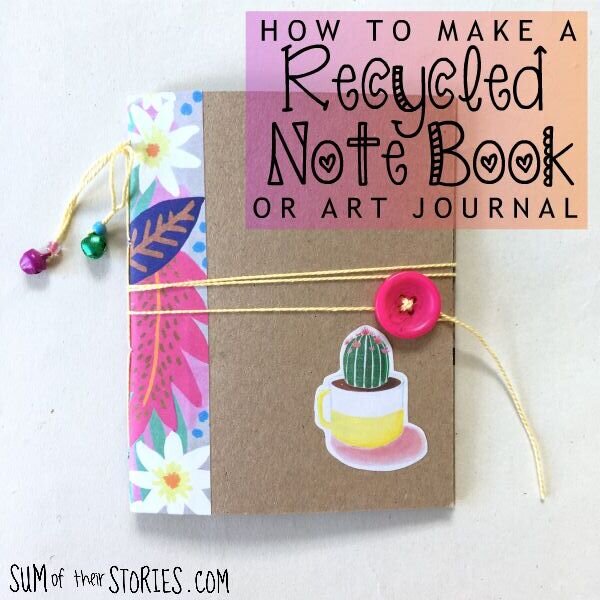The image is a square photograph designed for a how-to guide or blog article. It features a handmade notebook, created from recycled materials, displayed on a flat white surface. The notebook, with its brown cardboard cover, sits prominently in the center. It is bound on the left-hand side with a floral-patterned paper adorned with vibrant blue and pink leaves and white flowers. A thin, white twine encircles the notebook and is fastened with a small pink button on the cover. Additional decorative elements include a sticker of a yellow and white coffee mug with a green cactus sprouting from it, adorned with pink flowers, resting on a pinkish coaster. Overlaying the bottom of the image is black text reading "someoftheirstories.com," while the top right corner features a semi-transparent pink and purple rectangle with black text that reads "How to Make a Recycled Notebook or Art Journal."